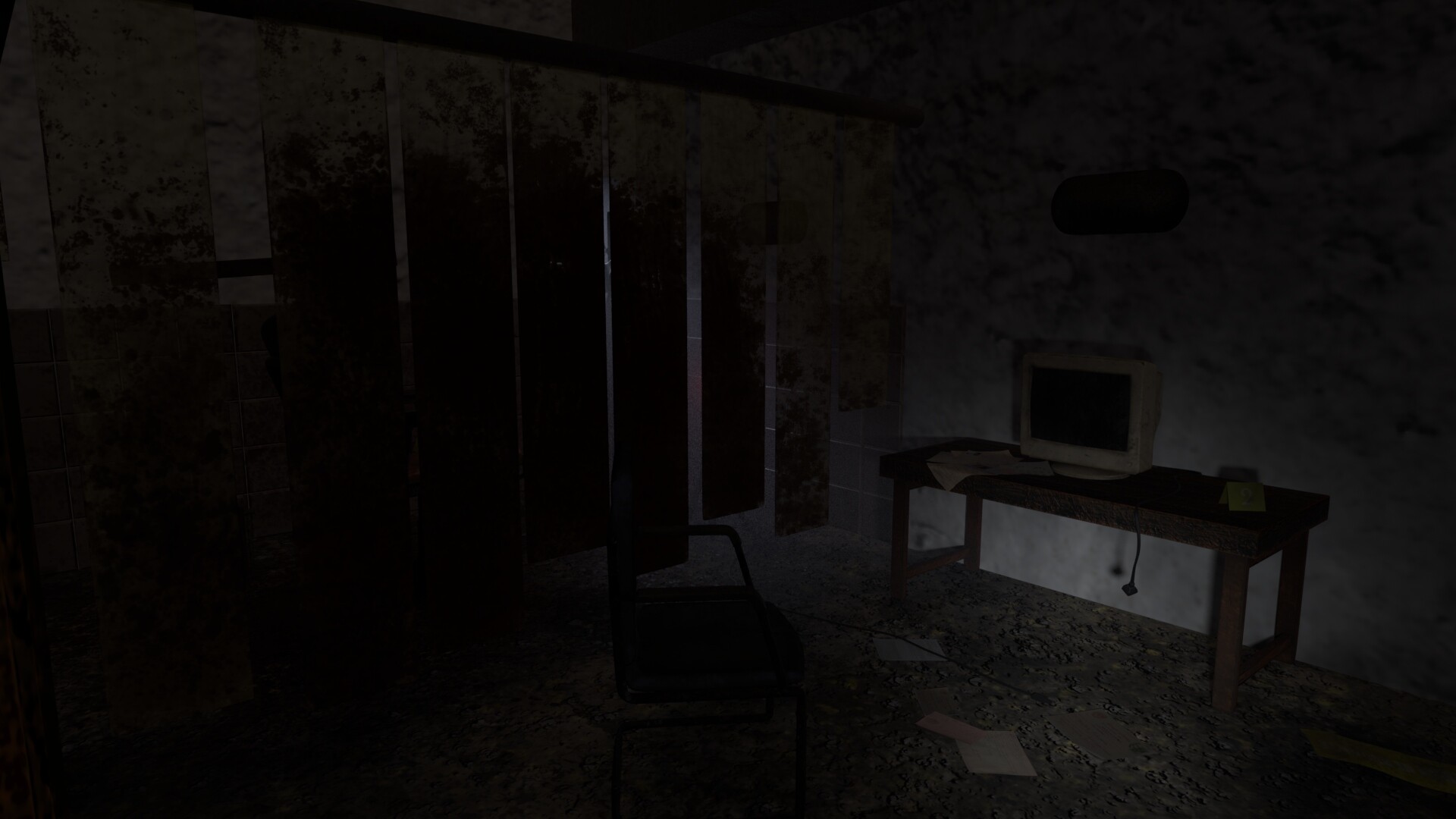The image depicts an extremely dark room, seemingly taken at night without any lights or flash. On the left side, which is almost entirely black, there's a discernible outline of either a window or a sliding door. Strips, perhaps drapes, hang from the ceiling with faint light seeping through them. The center of the photo suggests some ambient light sources, but details are hard to distinguish. 

The right side of the room is slightly more illuminated, revealing a grey wall and a small wooden desk or coffee table. Atop the table sits an old-style computer monitor with a white object draped over its edge and an electrical cord hanging down, casting a faint shadow against the wall. Scattered on the dark, possibly grey rug beneath are what appear to be papers. There are also rectangular-shaped mirrors reflecting minimal light against the back wall. Despite the sparse light, the overall impression of the photo is one of a dim, cluttered interior space.